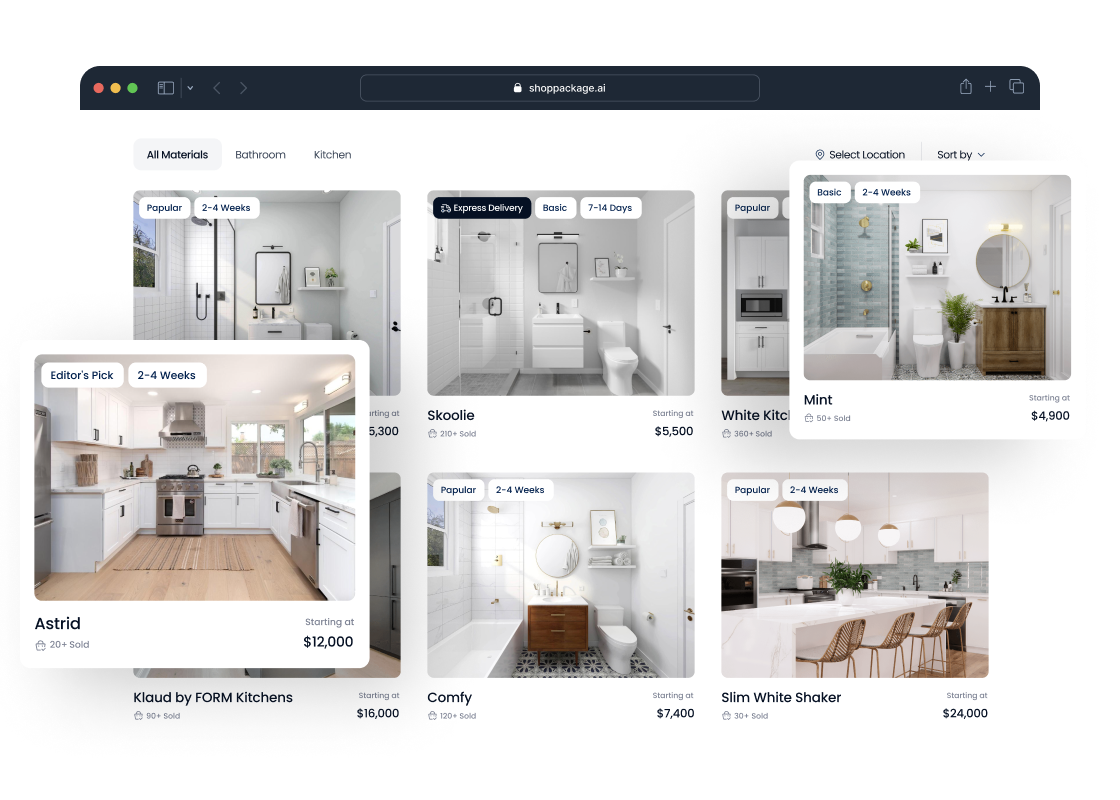The image is a horizontal rectangular layout featuring a distinct and organized design. At the top, there is a solid black bar stretching from left to right with a search bar that includes the text "Shop," although the rest is too small to decipher. Below the black bar, the main content area has a white background.

On the top left of this white background, there are three horizontally aligned rectangular labels. The first label is in bold black font and reads "All Materials." The next two labels are in regular black font and read "Bathroom" and "Kitchen," respectively. To the top right are dropdown menus labeled "Select Location" and "Sort By."

The image includes two rows of three pictures each, displaying various interior design layouts. There are two pop-ups overlaying some of these images. The top row initially features two images of bathrooms, whereas the third image is obscured by a pop-up, also showcasing a bathroom. 

In the bottom row, the first two images are of kitchens. A pop-up overlying the second image reads "Cloud by Form Kitchens," partially covering another kitchen image. The third image in this row is a bathroom.

The pop-up on the right mentions "Editor's Pick" in white text inside a white oval located at the top left corner, alongside another white oval indicating "Two to Four Weeks." This specific layout is named "Astrid" and is priced at $12,000. Several images have a "Popular" tag in the upper left corner where the "Editor's Pick" tag appears, along with the respective delivery time frames. Most of these indicate a shipping window of "Two to Four Weeks," except for the second image from the left, which states "Seven to Fourteen Days."

Each image in these rows is labeled with a unique style name, such as "Schooly," "Mint," and "Slim White Shaker," along with their respective prices.